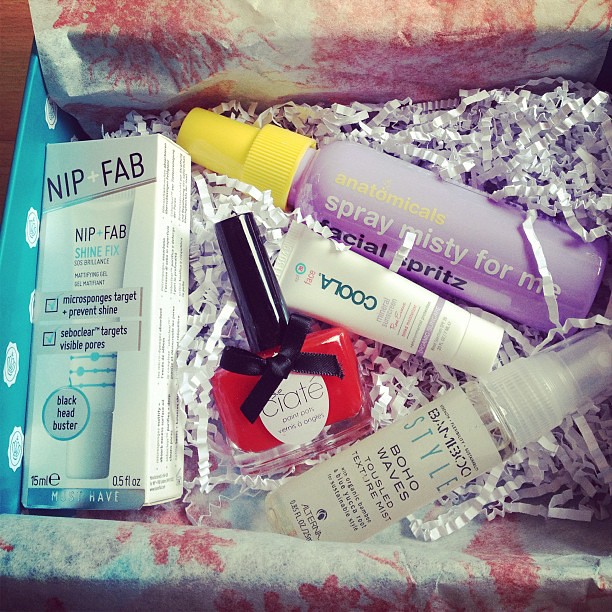In this detailed image, a recently opened gift or subscription box sits on a wooden table, brimming with decorative crinkly paper in white and hints of purple. Nestled within the paper are five distinct cosmetic products. On the left side, there's a rectangular black box labeled "Nip+Fab Shine Fix," a product designed for addressing blackheads. Adjacent to it, there's a vibrant red nail polish with a black cap labeled "Ciaté." A white squeeze tube, partly obscured and difficult to decipher, displays the brand "Coola," suggesting it might be a face cooler. A striking purple spray bottle with a yellow cap, named "Anatomicals Spray Misty For Me," offers a refreshing facial spritz. Lastly, a clear spray bottle with a white label identified as "Bamboo Style Boho Waves" promises to create textured, beachy waves. The entire presentation is thoughtfully cushioned with white and purple tissue paper, emphasizing the care taken in packaging these skincare and beauty products.